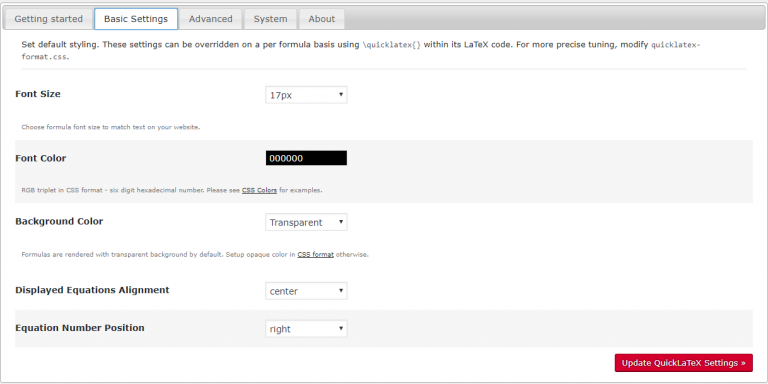The website interface displays five tabs at the top, each with light grey backgrounds and black text. The tabs are labeled as follows from left to right: "Getting Started," "Basic Settings," "Advanced," "System," and "About." The "Basic Settings" tab is currently selected, as indicated by a blue rectangle around its label.

Below the "Basic Settings" tab, there is a section titled "Set Default Styling," which includes the note: "These settings can be overridden on a per-formula basis using \quicklatex with its LaTeX code. For more precise tuning, modify quicklatex-format.css."

The settings adjustable within this section include:

1. **Font Size**: The current setting is 17 pixels.
2. **Font Color**: Displayed as a black box with the hexadecimal color code "000000" in white text inside it.
3. **Background Color**: Set to transparent.
4. **Display Equations Alignment**: Set to center.
5. **Equation Number Position**: Set to right.

At the bottom right corner of the page, there is an "Update QuickLaTeX Settings" button.